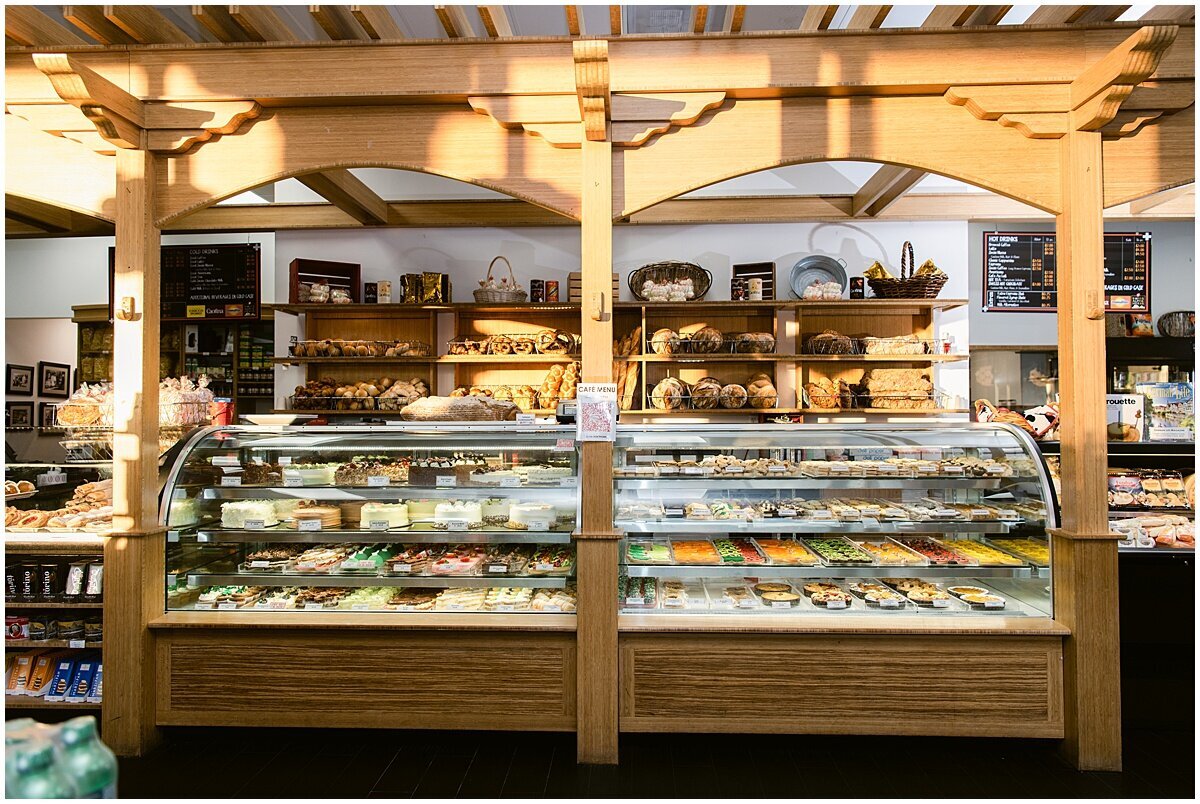This color photograph captures the intricate interior of a charming bakery. The focal point is a large glass display case with a rounded top, framed elegantly by wooden beams—three in total, positioned on the left, center, and right—that support a rustic wooden roof or pergola structure. The display case is filled with an assortment of cakes, pastries, and other confections, though the specific types are difficult to distinguish in detail. To the left side of the case are cakes and a variety of pastries, while the right side features a mix of baked goods and possibly cookies or other savory items.

Behind the display counter, wooden shelves line the white back wall, stocked with an array of bread items, including bagels, circular loaves, boules, and pretzels. The uppermost shelves are adorned with decorative items such as wooden crates and woven baskets. On the back wall, a chalkboard-style menu board, though too small to read, adds to the quaint ambiance. 

Adding to the detail, there is a café menu sign prominently placed on the center of the bakery counter, indicating the availability of additional offerings. To the left, lower shelves possibly display chocolate bars, and beyond that, hanging pictures and shelves with further displays contribute to the cozy interior. A door or passageway is also visible on the left, leading to another section of the store. The scene is devoid of any people, allowing the viewer to fully appreciate the warm and inviting setup of this delightful bakery.